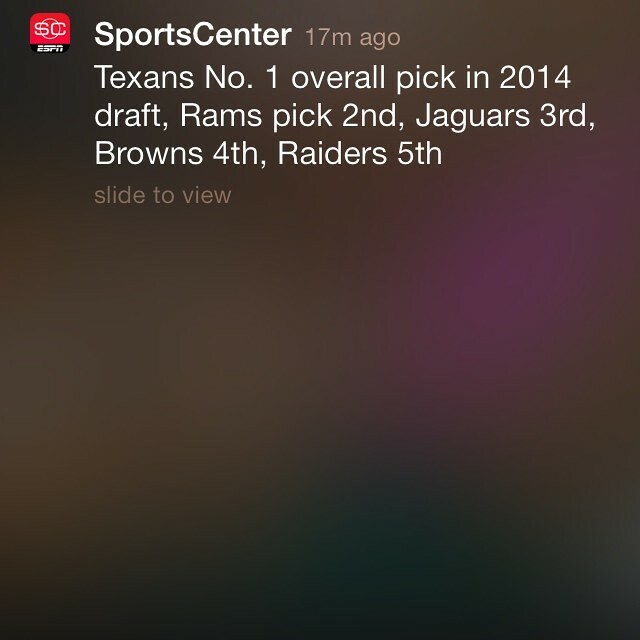This image depicts a notification from the SportsCenter app by ESPN on a phone lock screen. The notification, sent 17 minutes ago, reads: "Texans number one overall pick in 2014 draft, Rams pick second, Jaguars third, Browns fourth, Raiders fifth." The text, which provides details about the top five draft picks for the upcoming 2014 NFL draft, is prominently displayed in white with some brownish hues. In the top left corner, there is a small SportsCenter ESPN logo, featuring red and black elements with white text. The background of the screen is mostly brown with subtle hints of purple, giving it a slightly blurred and indistinct effect, reinforcing the focus on the notification itself. This setup resembles the style of a typical lock screen notification for users subscribed to SportsCenter updates.